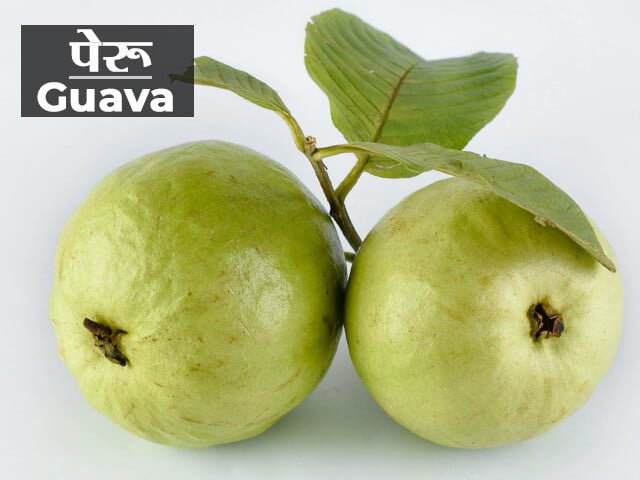The image features two spherical, green guavas centered against a light grey background. The guavas are attached to each other by a small brownish-black branch, which extends into three green leaves. One leaf bends backward while the others extend to the left and right. The guavas exhibit occasional brown spots. In the upper left-hand corner of the image is a semi-transparent dark rectangle with white text. The text reads "Guava" in English, with the 'G' capitalized, and above it, there is a line of foreign text, possibly in an oriental or Russian script. The detailed pattern of veins is visible on the leaves.